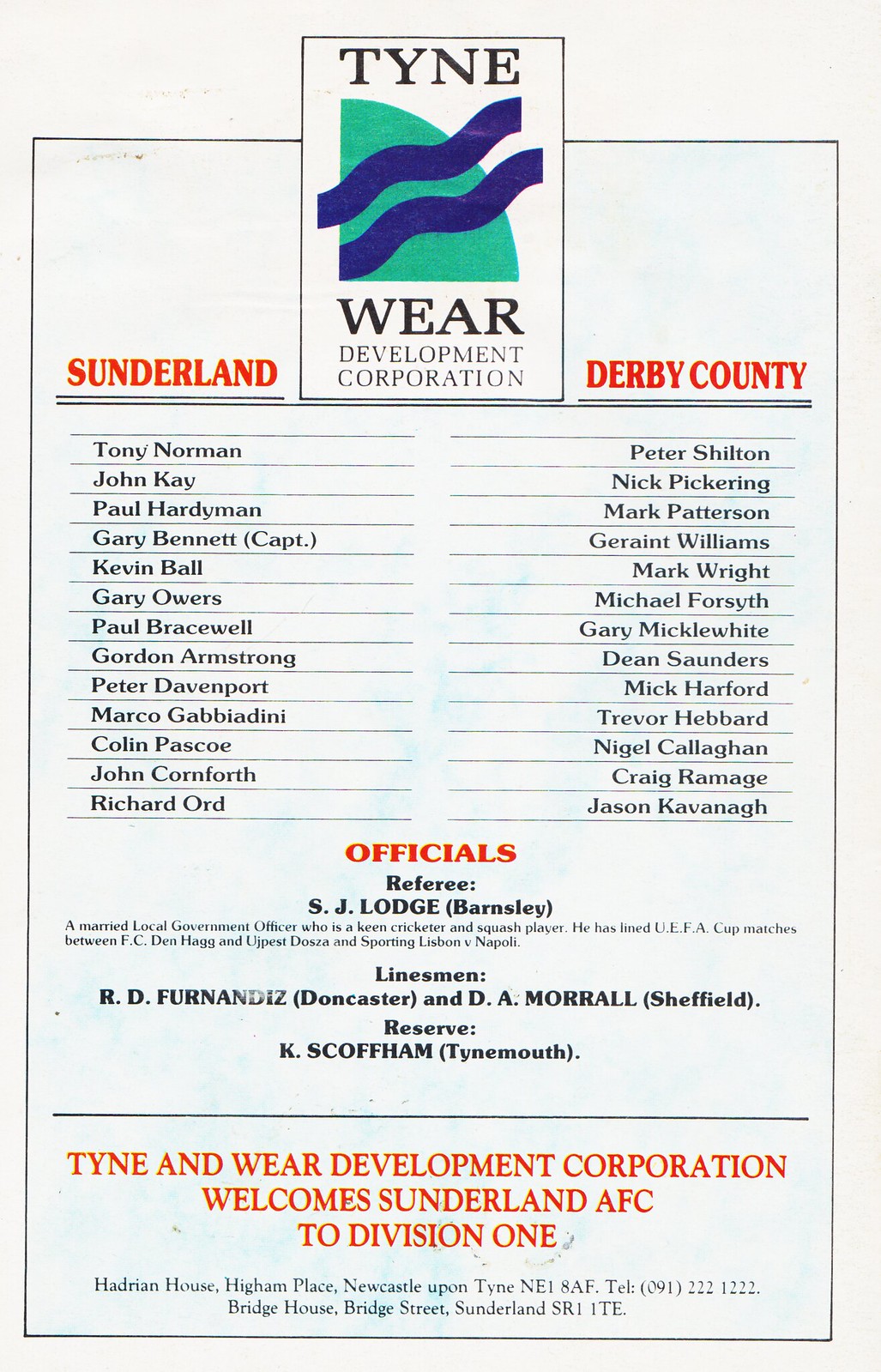This image depicts a page from a sports program, likely related to soccer or possibly rugby or cricket, given its English origin. The document appears on a white, bluish piece of paper. At the top center, enclosed in a box, it reads "Tyne" with the Tyne and Wear Development Corporation logo directly beneath it. The logo, featuring "W-E-A-R" in black lettering, is followed by "Development Corporation" in smaller print. On the left in red is the word "Sunderland," and on the right, it says "Derby County," suggesting the two competing teams.

The list comprises 26 names of players, split evenly between Sunderland on the left and Derby County on the right. Below the players' names, there is a section titled "Officials" in red text. In black below that, it lists:
- "Referee: S.J. Lodge (Barnsley)"
- "Linesmen: R.D. Furnandiz (Doncaster) and D.A. Moral (Sheffield)"
- "Reserve: K. Scoffham (Tynemouth)"

A dividing line follows, beneath which it states in reddish print, "Tyne and Wear Development Corporation welcomes Sunderland AFC to Division 1." Below this, the addresses and contact information for the Corporation are provided:
- "Hadrian House, Hyam Place, Newcastle upon Tyne, NE1 AF. Tel: (091) 222-2222"
- "Bridge House, Bridge Street, Sunderland, SR1 TE."

This detailed description encapsulates key information conveyed in the image with emphasis on repetitive and shared details.